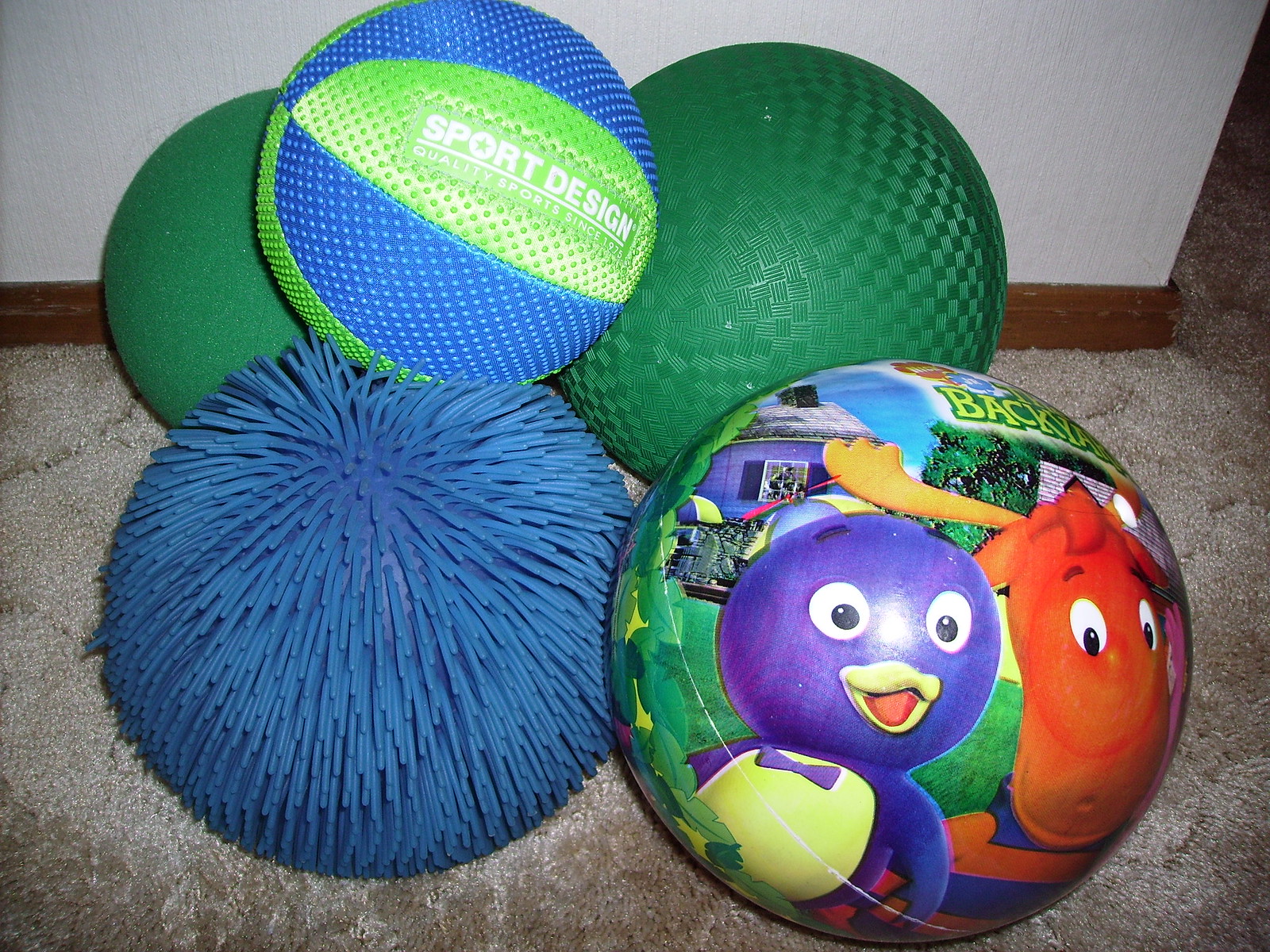This is an image of five large rubber balls stacked up against a white wall with brown wooden baseboard molding. The balls rest on a tan-colored carpet. Arranged in a triangular formation, the bottom row consists of four balls, and one sits atop them. 

In the back row, the two green balls vary in texture: the left one has a felt-like surface while the right has a shimmery checkered pattern, resembling a classic bouncy ball. In front of the felt green ball, there is a royal blue koosh ball with plastic tendrils extending from it. To its right, there's a ball featuring characters from The Backyardigans—a purple penguin wearing a propeller hat and an orange moose—predominantly in blue, green, and red colors. Perched on top of these four is a basketball with a dotted texture, bearing the inscription, "Sports Design, Quality Sports since 1975," in blue and lime green tones.